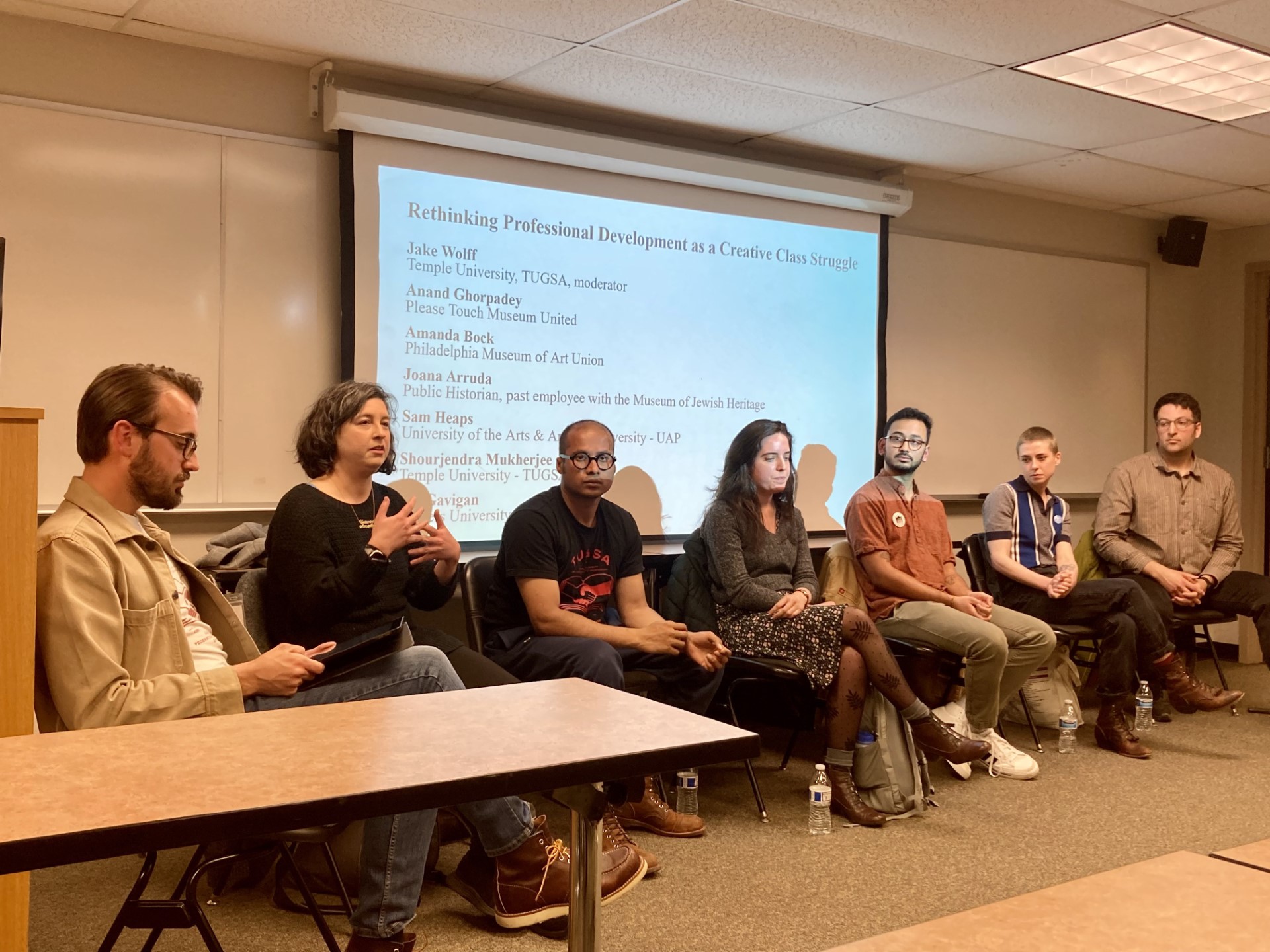The image captures an indoor scene at a conference or classroom panel discussion. In the foreground, several people are seated in chairs, engaged with an audience. On the far left, a man dressed in denim jeans, brown boots, an open jacket, and a t-shirt is holding a few black clipboards while looking down, possibly reading something. To his right is a woman clad in a long-sleeved black shirt and a necklace, her grayish-black hair framing her face as she gestures with her hands, indicating she is speaking. To her right, a man wearing glasses stares out at the audience attentively.

In the background, a projector screen displays the title of the session: "Rethinking Professional Development as a Creative Class Struggle." Underneath, the slide lists the names of the speakers and their affiliations. The participants include Jake Wolfe from Temple University TUGSA, moderator Aned Gorpathy, Amanda Bach from the Philadelphia Museum of Art Union, Jonna Arruda, the public historian and former employee at the Museum of Jewish Heritage, and Sam Heaps from the University of Arts UAP. Additional names such as Shor Jenda and Muk Girji are also visible, though one last name, Gavigan, is partially unreadable. The setting includes a carpeted floor and a table in front of the participants, adding to the formal yet relaxed atmosphere of the event.